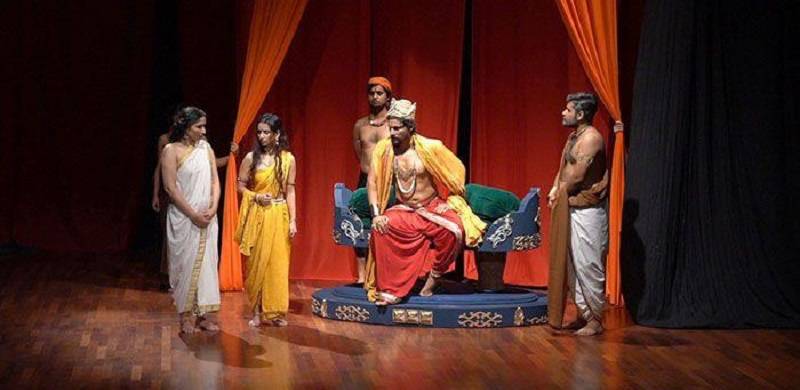This image captures a vibrant scene reminiscent of a Bollywood theatrical play or a richly-staged photo shoot. Five individuals, clad in elaborate costumes, are posed on a wooden stage framed by black and red drapes. To the left, two women stand elegantly. The woman closest to the edge is dressed in a white robe adorned with gold trim, which leaves one shoulder exposed. Her hands are delicately clasped in front of her body. Beside her, another woman wears a yellow robe, cinched at the waist with a belt, her long hair cascading over her shoulders and adorned with bands halfway up her biceps. 

At the center of the stage, a man exudes regal authority, seated on a blue platform that resembles a throne. He is dressed in a striking ensemble featuring red pants and an open yellow robe that reveals his bare chest, embellished with a necklace and a crown. A cuff wraps around his wrist, and an orange sash drapes over the back of his neck. Standing protectively behind him is a man with his arms tucked behind his back, wearing a red hat, a necklace, and black pants, but no shirt.

To the right of the central figure, another man observes the scene. He is adorned in a brown wraparound garment paired with white pants, his demeanor calm and composed. All characters are barefoot, emphasizing perhaps a traditional or historical narrative being portrayed. The wooden floor adds a touch of rustic authenticity to this visually captivating tableau.